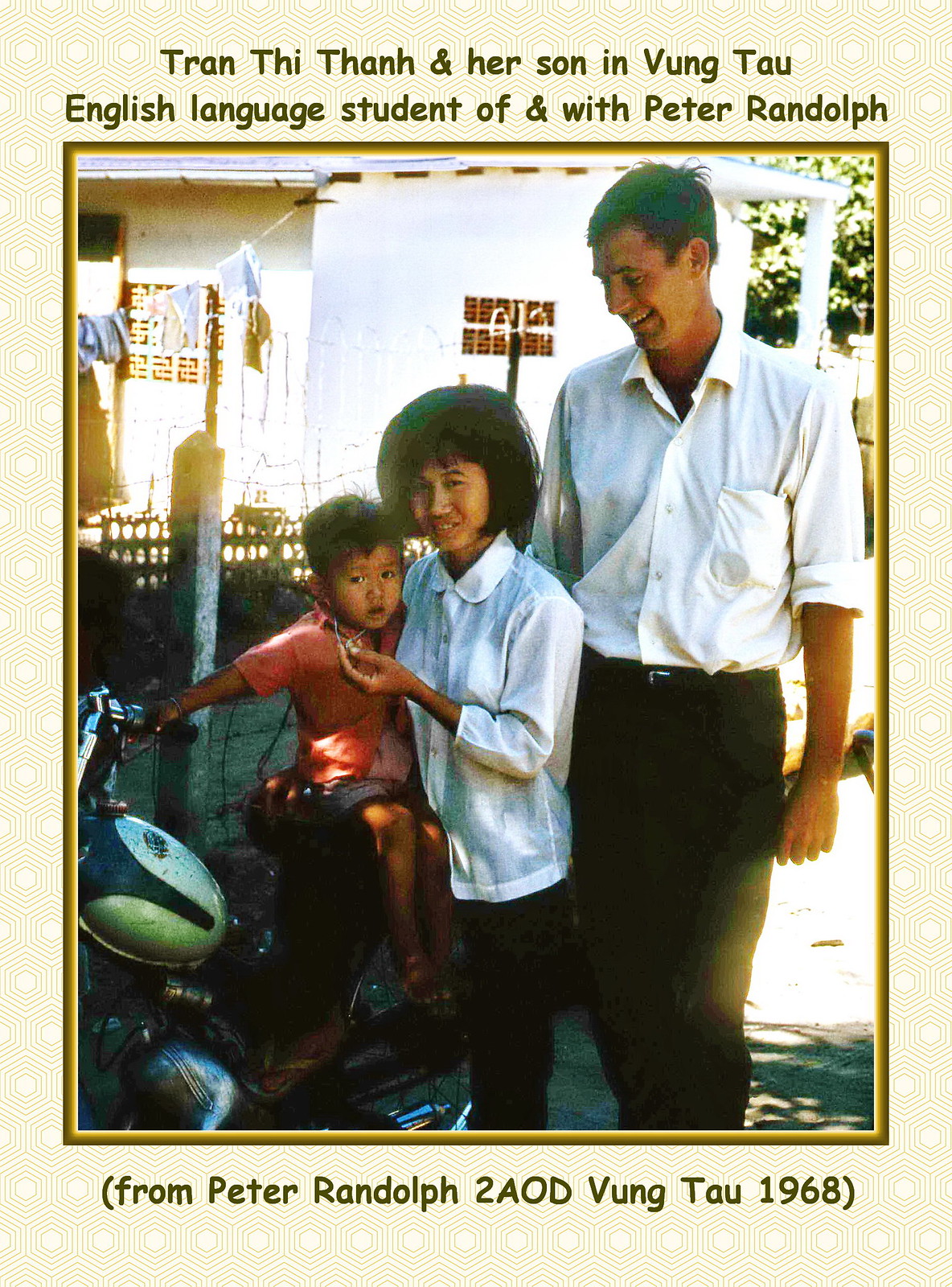This vintage photograph from 1968, set in Vung Tau, captures an intimate moment between three individuals. Dominating the right side of the image is a young Caucasian man, Peter Randolph, dressed in a white collared shirt with short-cropped hair and black pants. He gazes down affectionately at Tran Thai Tan, an Asian woman with thick black hair that curves down to her chin. She mirrors his attire with a white button-up collared shirt and black pants. Tran Thai Tan, smiling gently, holds her young son, who is perched on the seat of a burgundy motorbike with chrome handlebars. The boy, with short black hair, wears an orangey-red shirt and dark shorts, and is barefoot. Above the image, in black font over a light tan background, reads "Tran Thai Tan and her son in Vung Tau, English language student of and with Peter Randolph." Below the photo, a caption in parentheses states, "from Peter Randolph to a OD Vung Tau 1968."